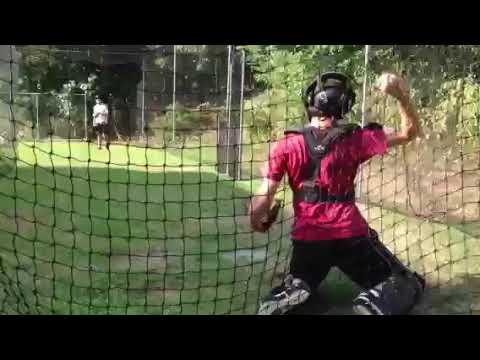The photograph features a daytime outdoor scene framed by black horizontal bars at the top and bottom. It is taken from behind a net resembling a soccer or goalie net. In the foreground, near the right side of the frame, a Caucasian boy is seen kneeling on both knees, dressed in a red short-sleeved shirt, black pants, and wearing protective gear including a black helmet, knee pads, and what appears to be a chest guard. His right arm is raised, holding a baseball, ready to throw, while his left hand sports a catcher's mitt. The grassy field stretches from right to left, with well-trimmed grass. In the distant background, a man in a white shirt and black shorts appears to be preparing to catch the baseball.